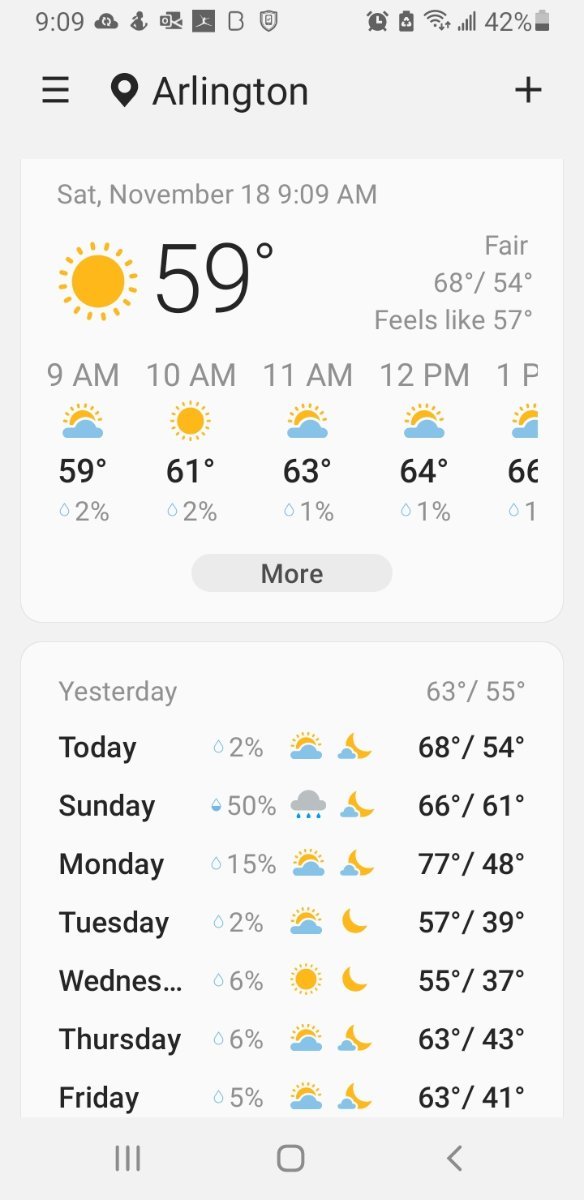The image displays a screenshot of a weather application on an iPhone, set to the location of Arlington. The specific state is not mentioned. The date shown is Saturday, November 18th, and the time is 9:09 a.m. The weather is marked by a sun icon, indicating clear conditions. The current temperature is 59°F, described as fair, with a high of 68°F and a low of 54°F. The "feels like" temperature is 57°F.

The app provides an hourly forecast for the subsequent hours: at 9 a.m. it is 59°F, 10 a.m. is 61°F, 11 a.m. is 63°F, 12 p.m. is 64°F, and 1 p.m. is 66°F. The chance of rain is minimal, around 2%.

Additionally, the app includes a weekly forecast, listing days from Sunday to Friday. The highest temperature in the upcoming week is forecasted to be 77°F on Monday, with a low of 48°F. Other days exhibit high temperatures averaging between 63°F and 68°F. This detailed layout is characteristic of a standard iPhone weather app interface.